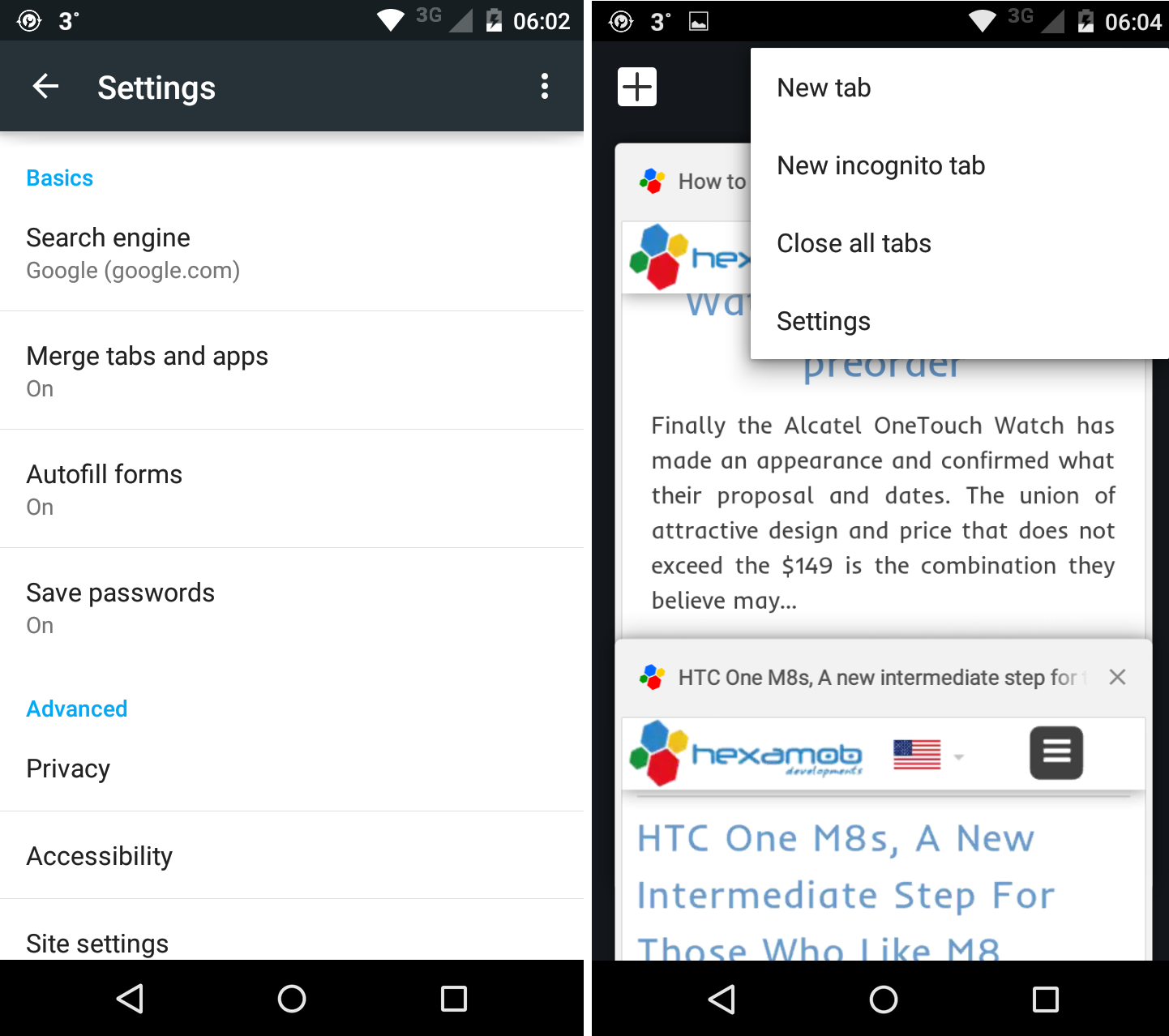This image captures two adjacent cell phone screens, juxtaposed to create a single comprehensive picture. 

On the left screen, a settings menu is clearly visible, beginning with a section titled "Basics." Within this section, the user’s default search engine is set to Google. Following this, there are various toggles indicating that "Merge tabs and apps," "Auto-fill forms," and "Save passwords" features are all enabled. The menu continues with an "Advanced" section, featuring further options such as "Privacy," "Accessibility," and "Site settings."

On the right screen, a browser tab open to a webpage called Hexa Mob is shown. A white pop-up menu is visible at the top of this screen, presenting options such as "New tab," "New incognito tab," "Close all tabs," and "Settings." Further down, the screen displays a snippet of text which reads: "Finally, the Alcatel OneTouch watch has made an appearance and confirmed what their proposal and date, what their proposal and dates. The union of attraction, design, and price that does not exceed the dollar or the $149 is the combination they believe may..." The text appears to be an excerpt from an article or a product review, abruptly ending in an ellipsis. 

Overall, the image details a side-by-side view of a phone settings menu and an active browser session, providing a glimpse into the user's device configurations and browsing activity.